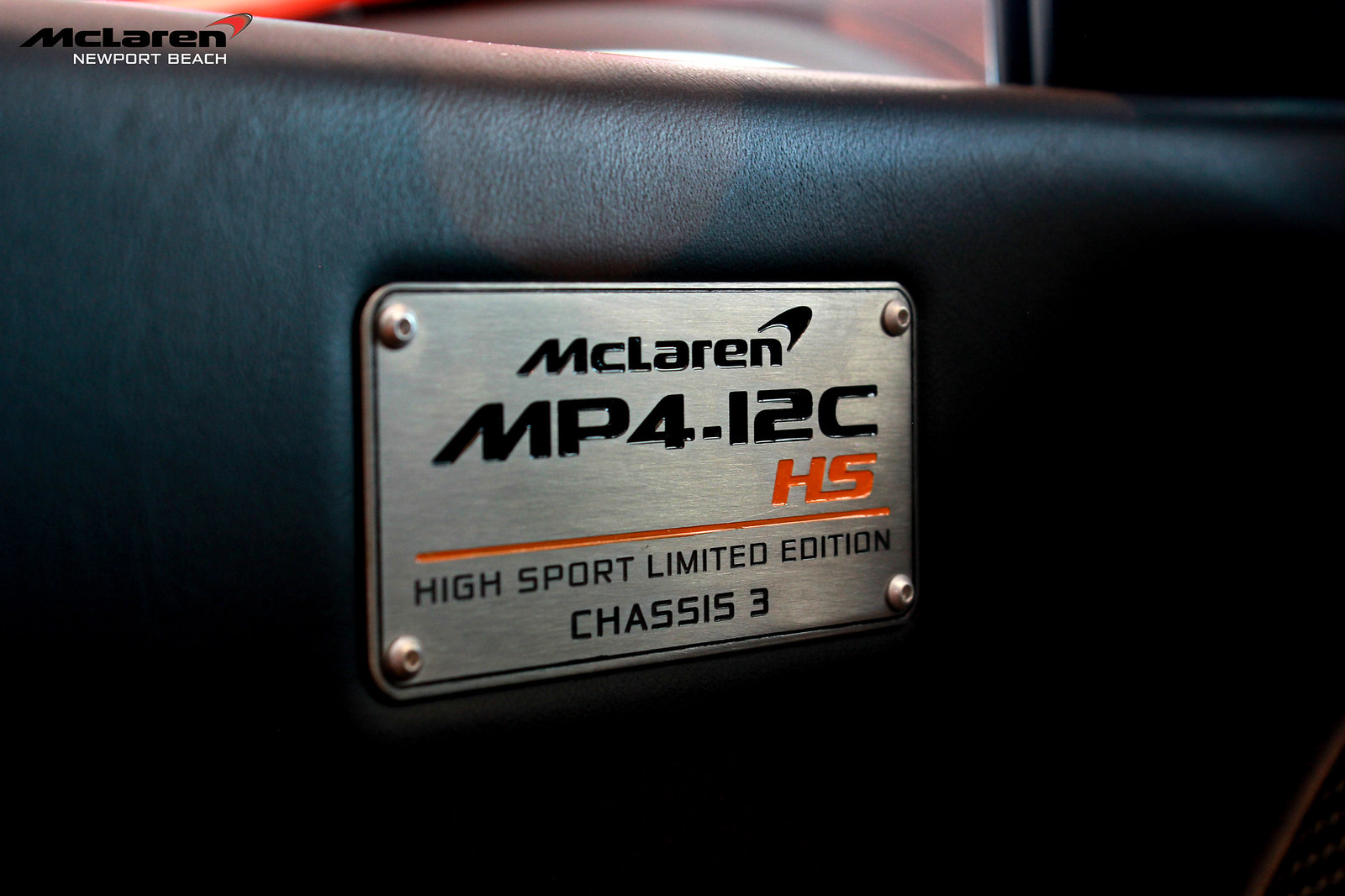The image depicts a close-up view of the luxurious black interior of a McLaren sports car. Prominently featured is a sleek black leather panel, which appears to be part of either the door or the seat. Attached to the leather is a steel plate with detailed inscriptions. At the top left of the plate, the McLaren logo is emblazoned in black, followed by "Newport Beach" in white text directly below it. Dominating the center of the plate, "McLaren MP4-12C" is written in bold black letters. To the bottom right, in striking red letters, the initials "HS" are displayed, accompanied by a red stripe running horizontally underneath. The final line of the plate features the words "High Sport Limited Edition Chassis 3" in black letters. This carefully angled photograph showcases the high-end craftsmanship and limited edition detailing of the McLaren MP4-12C HS.